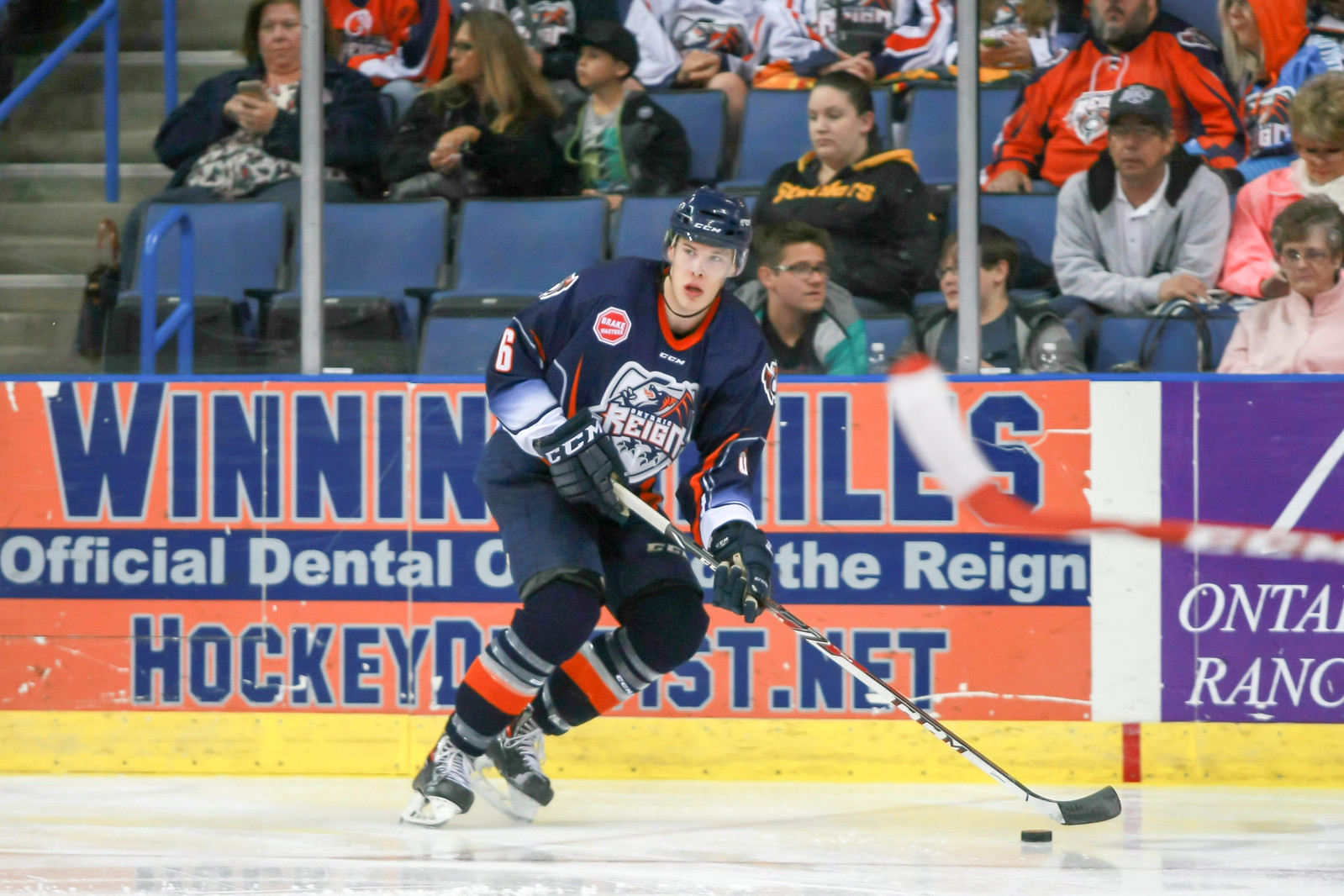The image depicts an intense moment in an ice hockey game, showcasing a player from the Ontario Reign, identifiable by his navy blue jersey with "Reign" emblazoned in white letters across the front. He is in action, stick in hand, maneuvering the puck across the rink's white ice. The player's gear features accents of red around the collar and on his skates, which also have red and blue detailing. He is poised towards the right, focusing intently on the puck that lies at the edge of his long white hockey stick, while looking off to the left.

Behind him, the rink's barricade prominently displays advertisements, including a large orange and blue one for "Official Dental Something The Reign," spanning from the left to beyond the middle. Further to the right is another purple advertisement. The tall plexiglass windows, framed by silver metal, ensure the spectators' safety as they enjoy the game from the blue-seated stands. The crowd fills most of the seats, though a few remain empty. In the upper right corner of the image, a set of gray cement steps with a distinct blue handrail leads to additional seating levels, further contextualizing the bustling hockey stadium environment.